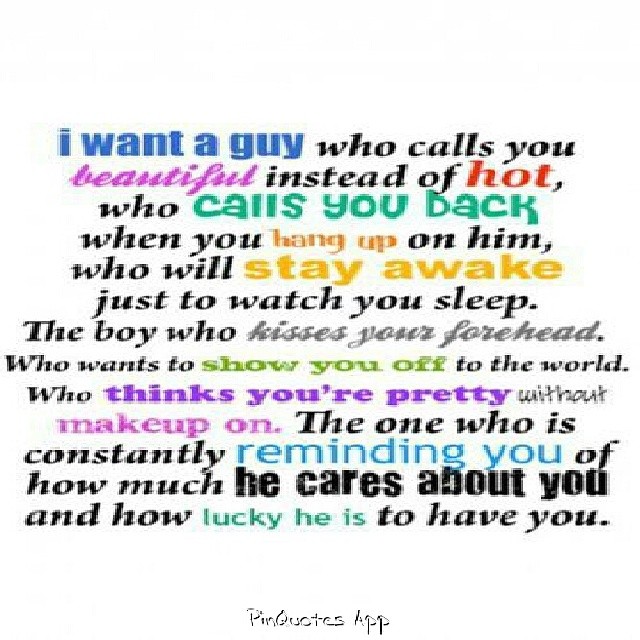This image consists of a detailed, multi-colored and multi-font text set against a white background. The quote reads: "I want a guy who calls you beautiful instead of hot, who calls you back when you hang up on him, who will stay awake just to watch you sleep. The boy who kisses your forehead, who wants to show you off to the world, who thinks you're pretty without makeup on, the one who is constantly reminding you of how much he cares about you and how lucky he is to have you." The text features various colors including dark blue, black, purple, red, teal green, orange, golden yellow, gray, olive green, and a lighter blue. The words "I want a guy" are prominently displayed in blue, while key words like "beautiful" and "hot" are highlighted in purple and red respectively, and different fonts are used throughout to emphasize the sentiment. At the bottom of the image, in lighter text, it indicates that it is from a "pin quotes app."